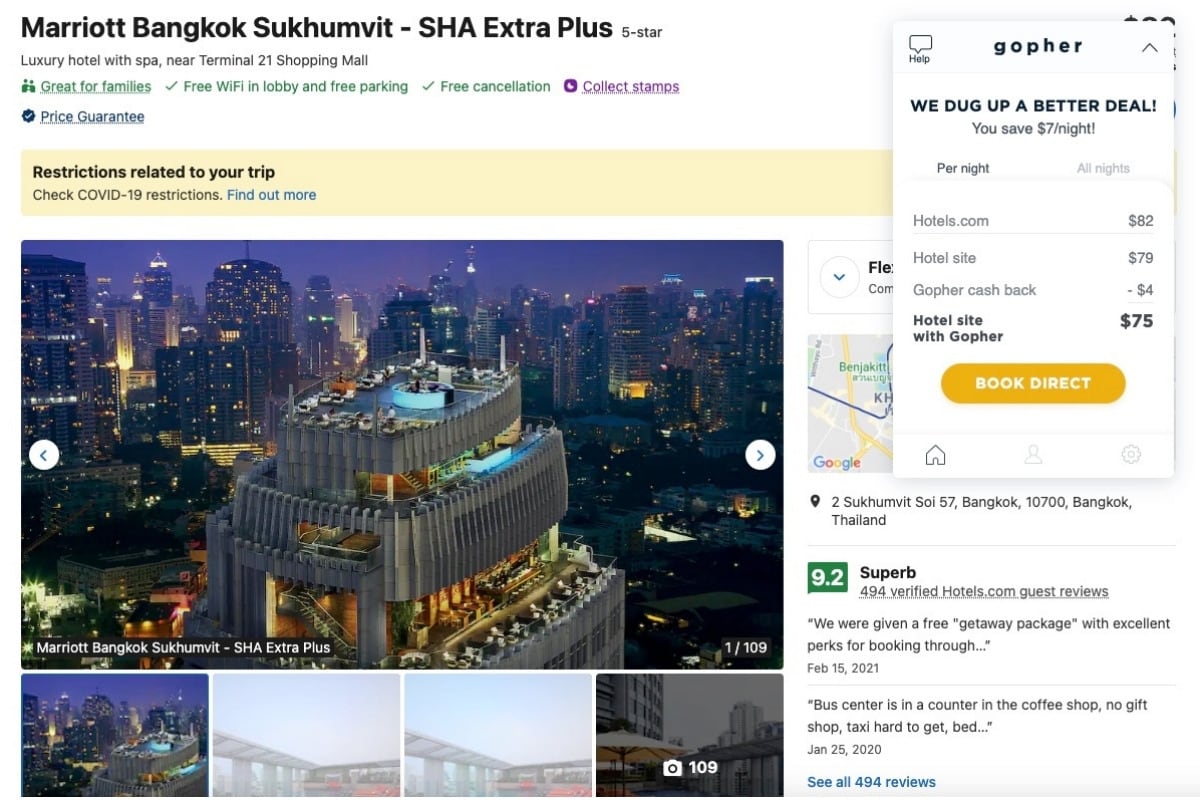The image caption, enhanced for clarity and detail, reads as follows:

**Marriott Bangkok Sepumbit-SHA Extra Plus**

In smaller letters beside the plus, it declares: *****5-star Luxury Hotel with Spa near Terminal 21 Shopping Mall. 

Below that, a green graphic depicts two icons representing people beside the words "Grateful Families." 

It also includes:
- **Free Wi-Fi in Lobby and Free Parking** 
- **Free Cancellation** (indicated with a checkmark)

Further down, a purple icon, possibly a phone, says **Collect Stamps**.

A seal with a checkmark reads **Price Guarantee**.

Below these, a light yellow banner stretches across the width of the image with bold text: **Restrictions Related to Your Trip**. In blue text, it advises: **Check COVID-19 Restrictions, Find Out More.**

Off to the right, a white rectangular pop-up appears. In the upper left corner of the pop-up is a help bubble labeled in lowercase bold letters, **gopher**. An up arrow next to it proclaims: **We Dug Up a Better Deal. You saved $7.00/night!** 

To the right of this, it concludes with the phrase **All Rights**.